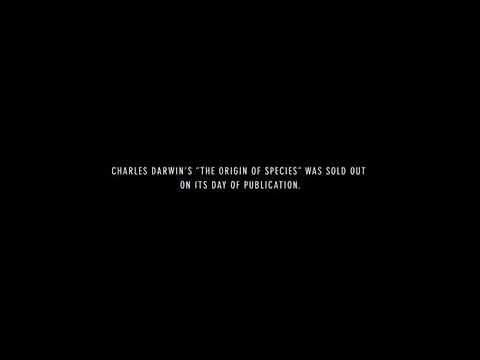The image is a perfectly square shape with a completely black background devoid of any artwork or design. At the center of the image, there is small, all-uppercase, white text. The text is succinctly displayed in two lines with ample space around it. The first line reads, "CHARLES DARWIN'S 'THE ORIGIN OF SPECIES' WAS SOLD OUT," followed by the second line, "ON ITS DAY OF PUBLICATION." This minimalist image serves as a factual message, highlighting the significant historical detail of the rapid success of Darwin's book on the day it was published.